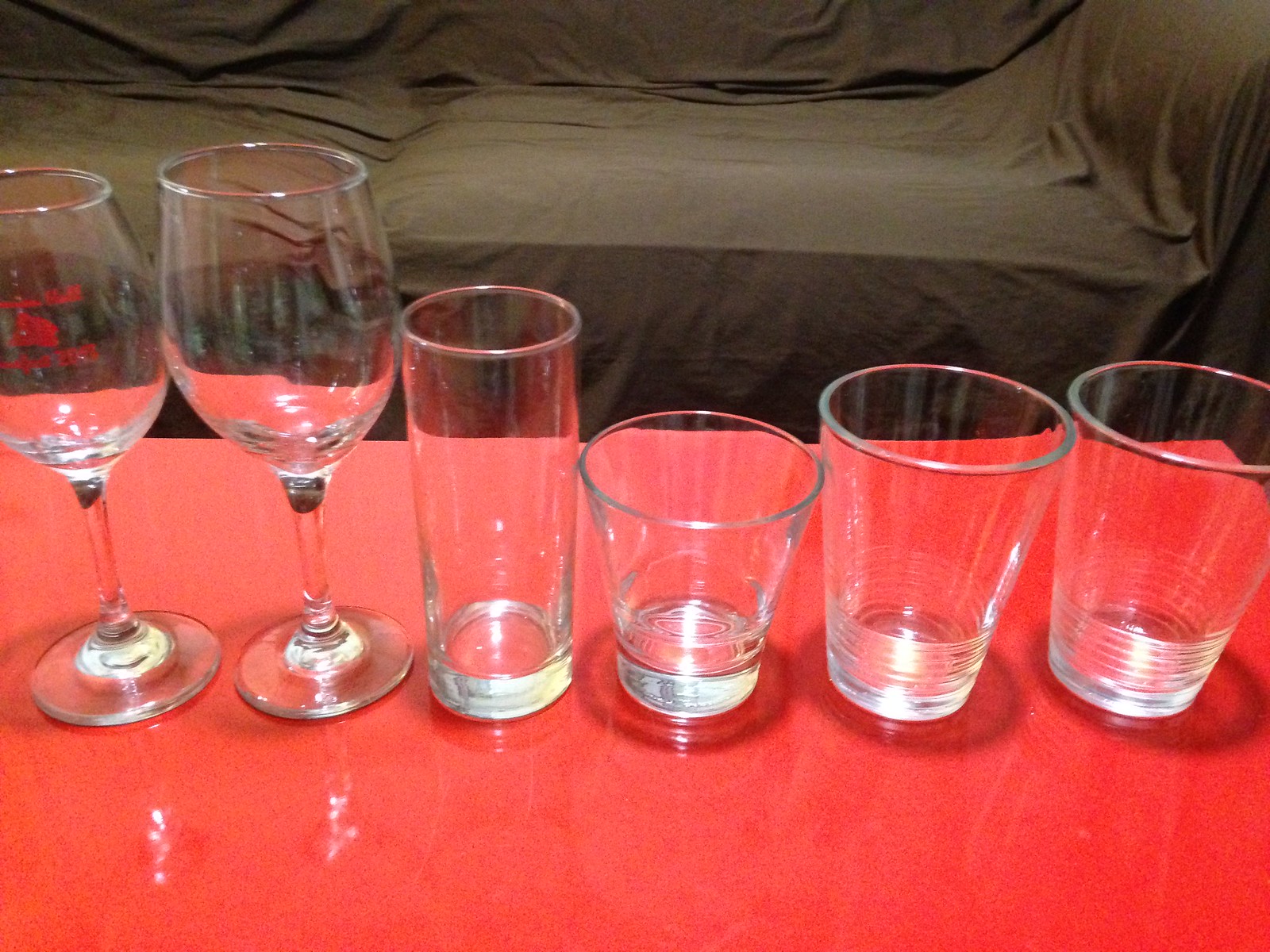This color photograph captures six clear glasses meticulously arranged on a high-polished bright red table. The glasses, which all appear to be empty, are positioned in a left-to-right sequence. On the far left, there's a wine glass with a narrower mouth that has some red, illegible writing on it. This glass's edge is slightly outside the picture's boundary. Adjacent to it is another, slightly larger wine glass. Beside the wine glasses stands a tall, thin tumbler, reaching about two-thirds the height of the wine glasses. Next in line is a shorter, fluted tumbler, similar in shape to a shot glass but broader. Further to the right, there are two slightly larger tumbler glasses that taper towards the bottoms and have fluted designs with noticeable lines or rings around their lower parts.

In the background, a couch draped with a crumpled, dark, brownish-green cover is visible, confirming the indoor setting. The light shines upon the glasses, causing reflections that highlight both the clear glass material and the shiny red table underneath. No additional objects are visible in the photograph, keeping the focus solely on the glassware arrangement and the covered couch.